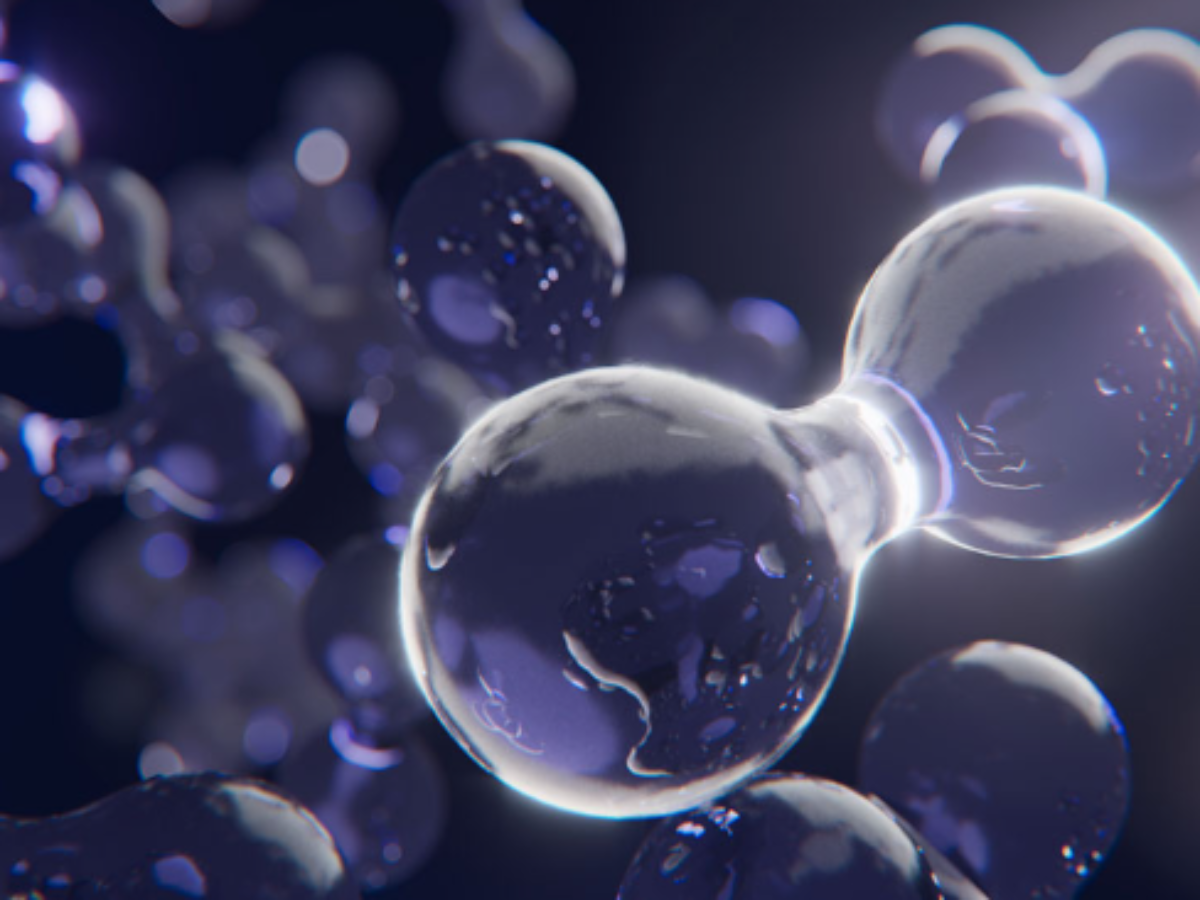This image presents an abstract depiction of several purplish orbs floating against a gradient background that transitions from black on the left to grey on the right. Dominating the foreground, there are two prominent spheres linked together, resembling an old-fashioned dumbbell. The central sphere, slightly below the center of the frame, is a deep purple with a lavender splotch on its bottom left and circled by a glowing white outline. This orb seamlessly merges into a similarly colored sphere on its right, connected by a thin strip resembling a liquid bridge between them. Encircling these primary spheres, the rest of the frame is filled with additional orbs that progressively blur as they recede into the background, creating a bokeh effect. The overall tone of the image is dark purple with reflective and glowing elements, suggesting a digital or AI-generated composition that evokes an ethereal and futuristic aesthetic. The spheres appear wet and highly reflective, adding to the mystical and abstract quality of the scene.